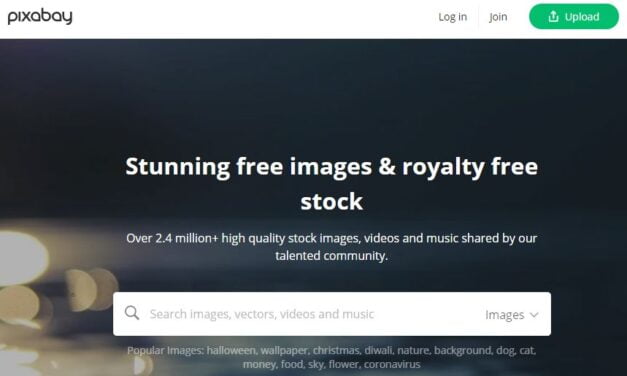Screenshot of the Pixabay Homepage: 

The screenshot showcases the homepage of Pixabay, a company offering royalty-free stock images. The company name "Pixabay," written in a sleek, modern black font that appears to drip downwards, prominently sits at the center. In the top-right corner, the options to "Login" and "Join" are available in grey font. Further to the right, there's a green "Upload" button featuring an upload icon, with the word "upload" displayed in white.

At the center of the page, bold text announces "Stunning free images and royalty-free stock," followed by a subtext highlighting "Over 2.4 million high-quality stock images, videos, and music shared by our talented community." Below this, a prominent search bar invites users to "Search images, vectors, videos, and music," with a drop-down caret allowing users to refine their search categories. 

The page suggests popular search terms such as "Halloween," "wallpaper," "Christmas," "Diwali," "nature background," "dog," "cat," "money," "food," "sky," "flower," and "coronavirus."

In the background, the image features a dark blue gradient with subtle lights peeking out from the bottom left. White and yellow reflections and beams of light stream across the bottom half of the screenshot, adding a dynamic and visually appealing backdrop.